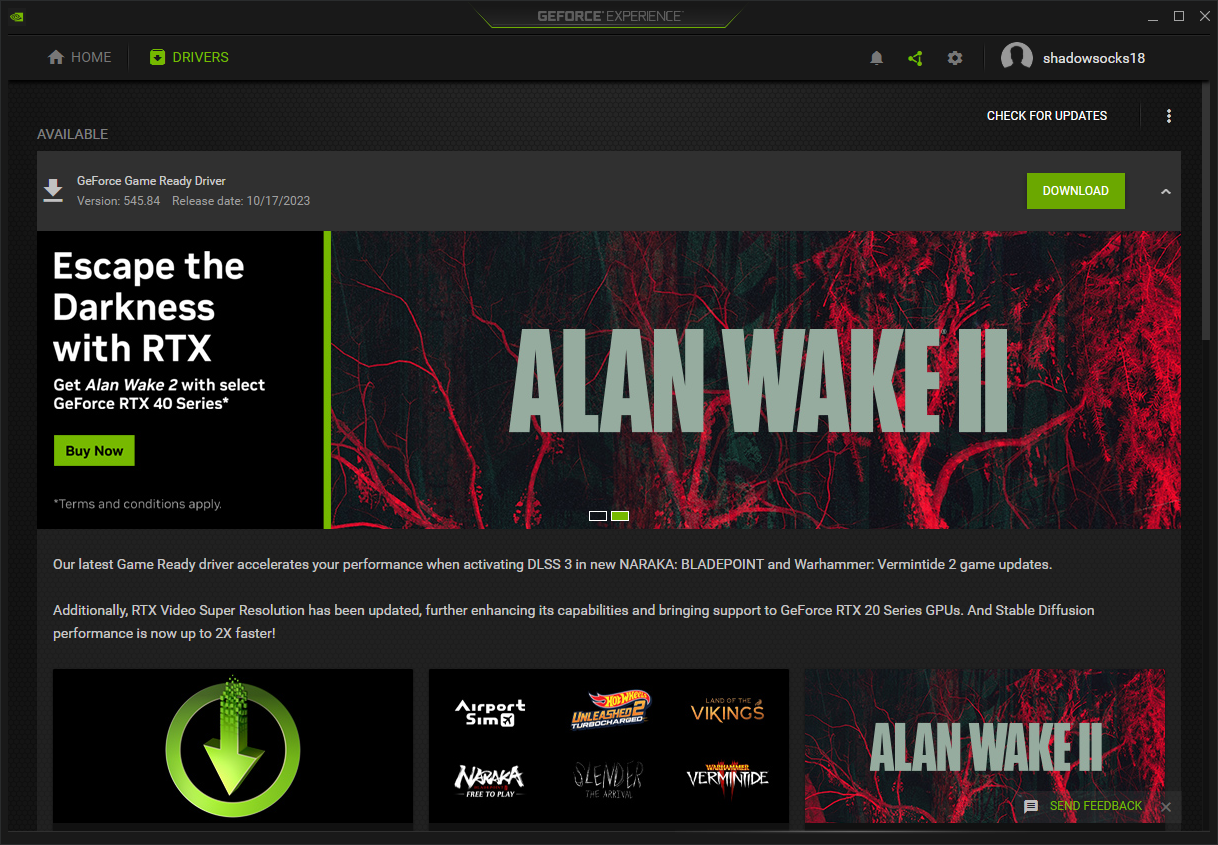The image depicts a dark-themed web page, predominantly black with accents of dark gray tones. At the top of the page, the title "GeoForce Experience" is prominently displayed, highlighted by a bright green underline. This green hue, distinctive and vibrant but not reminiscent of holiday shades, contrasts sharply with the darker background, drawing attention to key interactive elements.

In the central part of the image, the title "Alan Wake 2" is prominently featured. The background here is textured with the image of trees, dramatically illuminated by red lighting, adding a visually striking and atmospheric touch.

Navigational buttons are positioned at the top, with a "Home" button and a green-colored "Drivers" button. There is also a green "Download" button clearly visible. On the left side of the page, a "Buy It Now" button is similarly highlighted in green, ensuring it's easy to locate.

Emphasizing the title "Alan Wake," a long, skinny green rectangle runs vertically alongside it, enhancing its prominence. Completing the interface, the bottom left-hand corner showcases a green downward-pointing arrow encased within a green circle, signaling additional navigation or download options.

The combination of vivid green and bold red lighting not only enhances the aesthetic appeal but also effectively guides the user's attention across the web page.